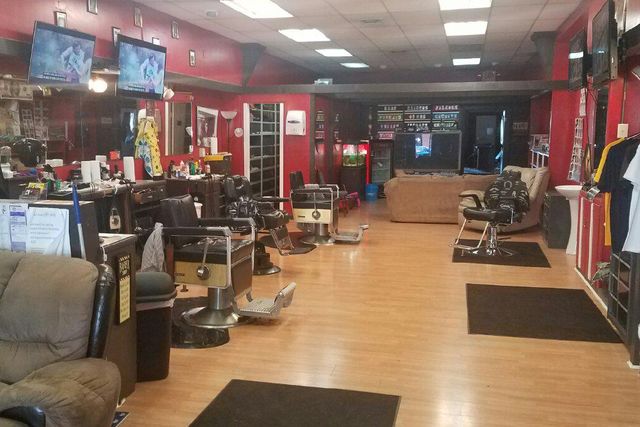The image showcases the interior of a contemporary barbershop with a vibrant and inviting aesthetic. The walls are painted a bold red, contrasting with the shiny wooden floor that is partially covered with three brown mats. Lining both sides of the shop are multiple barber chairs, suggesting a busy and functional space. Overhead, white fluorescent lights cast a bright, even glow across the room. 

In the background, a cozy seating area features a brownish-colored sofa and a recliner, providing a comfortable waiting space for customers. The shop is equipped with several flat-screen TVs, with at least two positioned near the barber chairs, possibly tuned to the same channel, catering to entertainment needs, likely sports given the overall masculine theme. Typical barbershop essentials such as brooms and garbage cans are also visible, adding to the authentic feel.

There is an area along one of the walls designated for hanging clothes, displaying t-shirts in various colors including black, yellow, and white. Although no people are present in the image, the setup indicates a well-maintained, ready-to-use barbershop that focuses on customer comfort and entertainment.